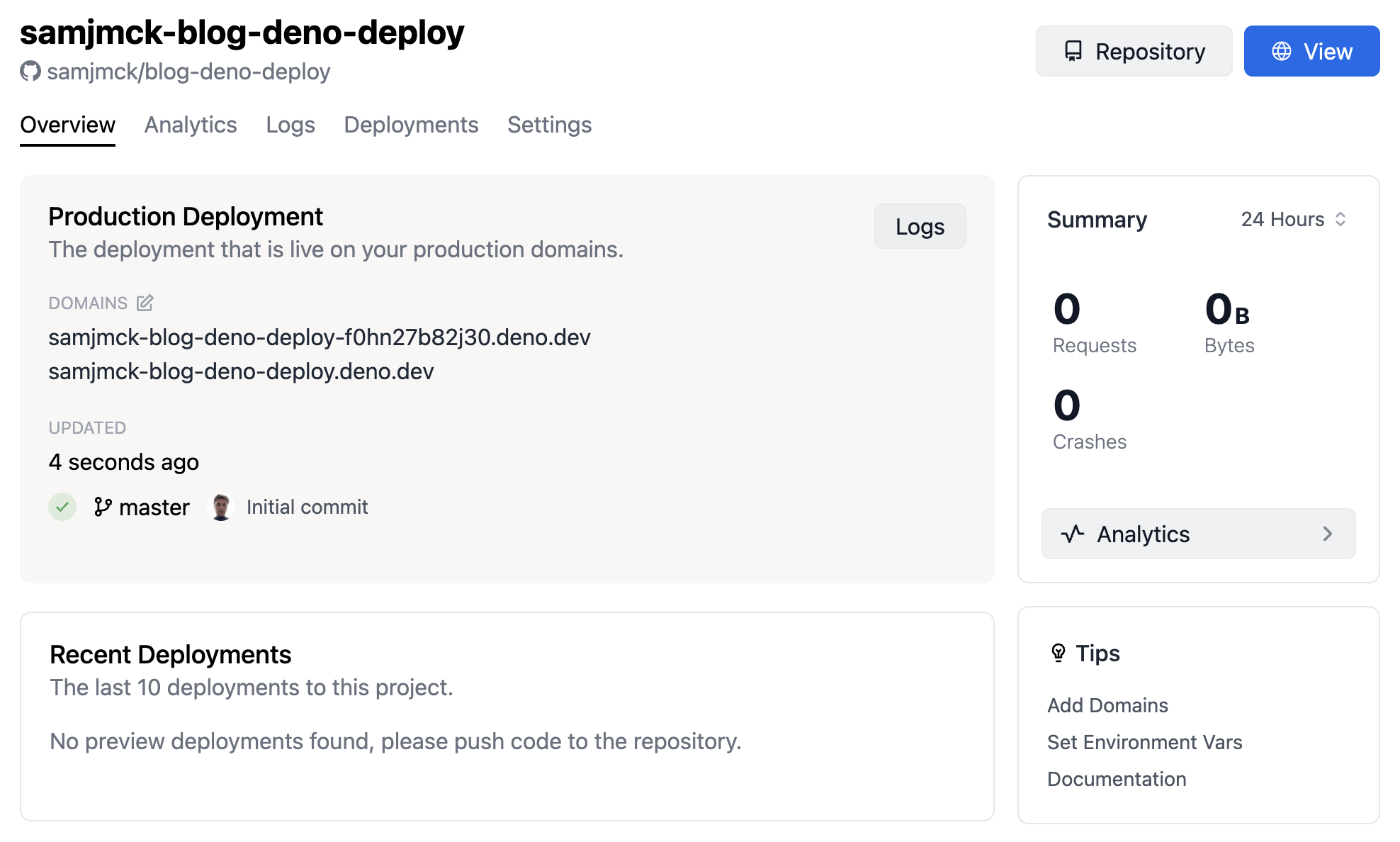This image captures the interface of a website dashboard, predominantly featuring a white background with various UI elements. 

At the top right corner, there's a blue button labeled "View" in white text, positioned next to a gray button with black text that reads "Repository." 

On the middle right, a small gray-outlined square contains a summary section indicating "Summary, 24 hours." Below this heading, it lists "0 requests," "0 B bytes," and "0 crashes." At the bottom of this square, a gray button inscribed with "Analytics" in black text, accompanied by a right-facing arrow, is visible.

At the bottom right, another small gray-outlined rectangle presents a white interior with the text: "Tips: Add domain, Set environment, VAERS documentation."

The top left corner of the site features the main text "samjmck-blog-deno-deploy" in bold, with a lighter gray repetition of the same text beneath it. Below this heading, five navigational tabs are visible: "Overview," "Analytics," "Logs," "Deployment," and "Settings." The "Overview" tab is bold and underlined.

A large, light gray rectangle below the tabs displays "Production Deployment." A gray button labeled "Logs" is positioned at the top right of this rectangle. An annotation beneath it specifies that the deployment is live on production domains, with the names of the domains listed and a note of the last update made "four seconds ago."

At the bottom of the page, a white rectangle outlined in gray reads "Recent Deployments: The last 10 deployments to this project." It also states "No preview deployments found. Please push code to the repository."

This detailed layout captures the comprehensive structure and key aspects of the website's dashboard interface.